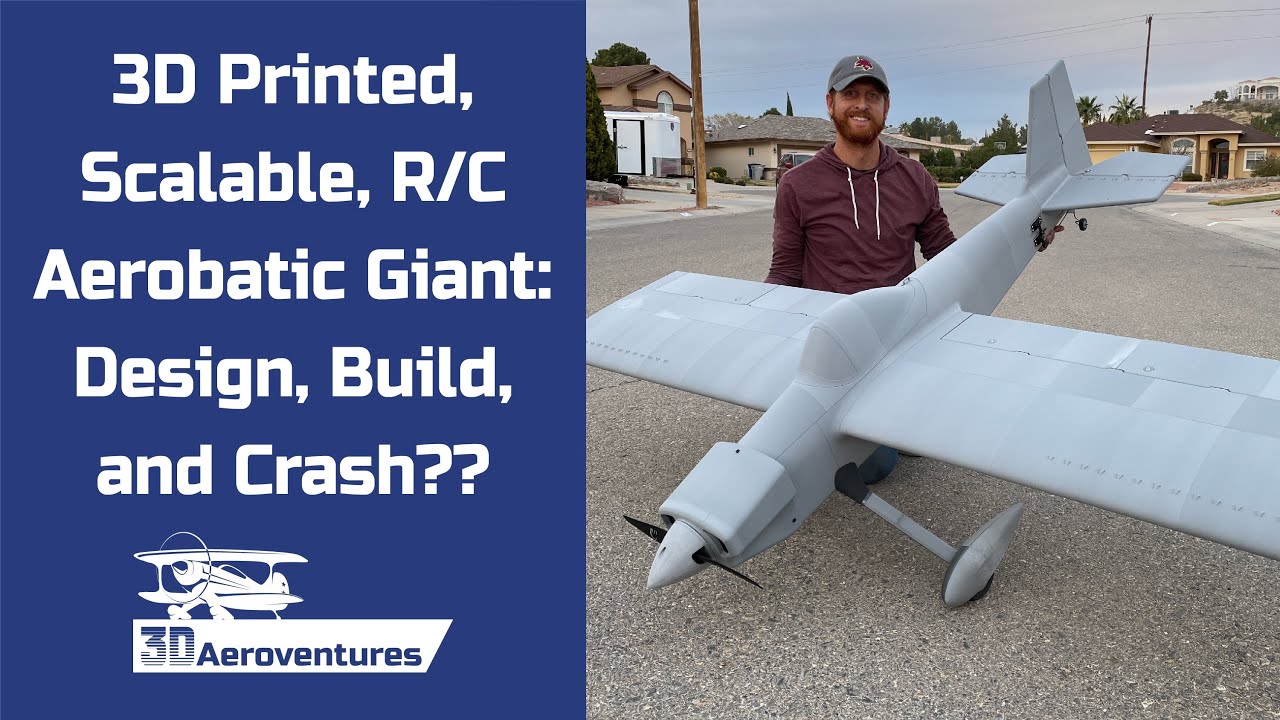The image showcases an advertisement for 3D Aero Adventures. The left side of the image features a royal blue panel with bold white text that reads: "3D printed, scalable, RC, aerobatic, giant, design, build, and crash??". Below this text, there is a logo of a white biplane with a dark blue banner underneath it stating the company name "3D Aero Adventures". The right side portrays a man standing on a suburban street, holding a large gray model airplane. This model airplane, which is bigger than the man himself, has its nose pointed downward while he grips the tail, elevating it. The man is seen from the front, wearing a maroon hoodie with white drawstrings and a gray cap. He has a dark brown beard and mustache. The background reveals a suburban street with houses and possibly a telephone pole, under a sky fading from light blue to gray.